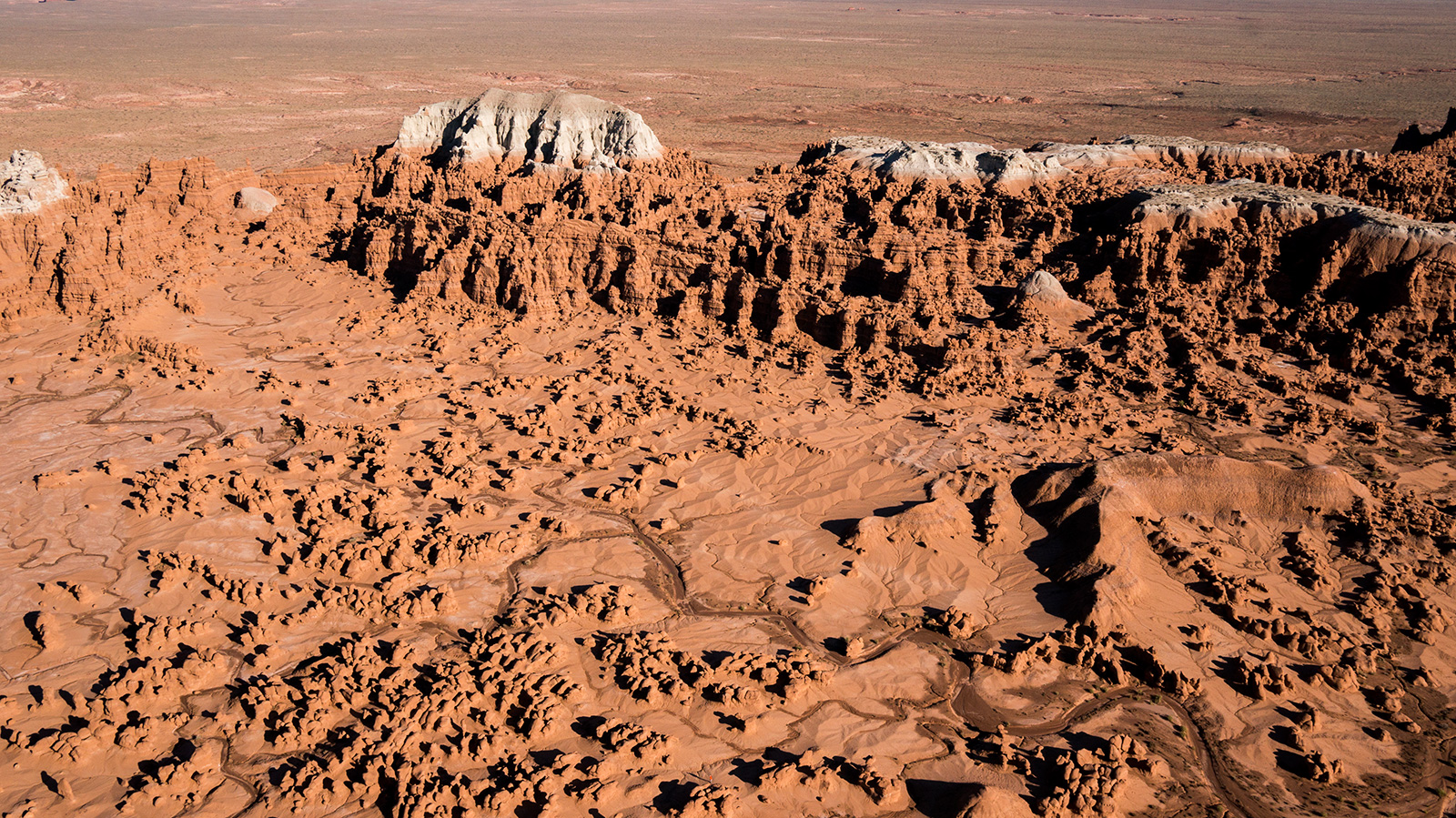This image captures an expansive, rugged landscape reminiscent of the Grand Canyon, dominated by vast expanses of dark red clay. The earth appears weathered and eroded, creating numerous divots and craters across the terrain. The ground is textured with rocky and sharp areas, forming uneven hills and lower regions. These hills vary in size from small mounds to larger formations, with some topped by patches of white or gray stone, adding stark contrast to the predominant red hues. The scene is entirely devoid of greenery or shrubberies, emphasizing its arid and desolate nature. The unique red-orange clay and the intricate patterns carved by natural forces suggest old, dried riverbeds that once weaved through this stark, vibrant desert landscape.